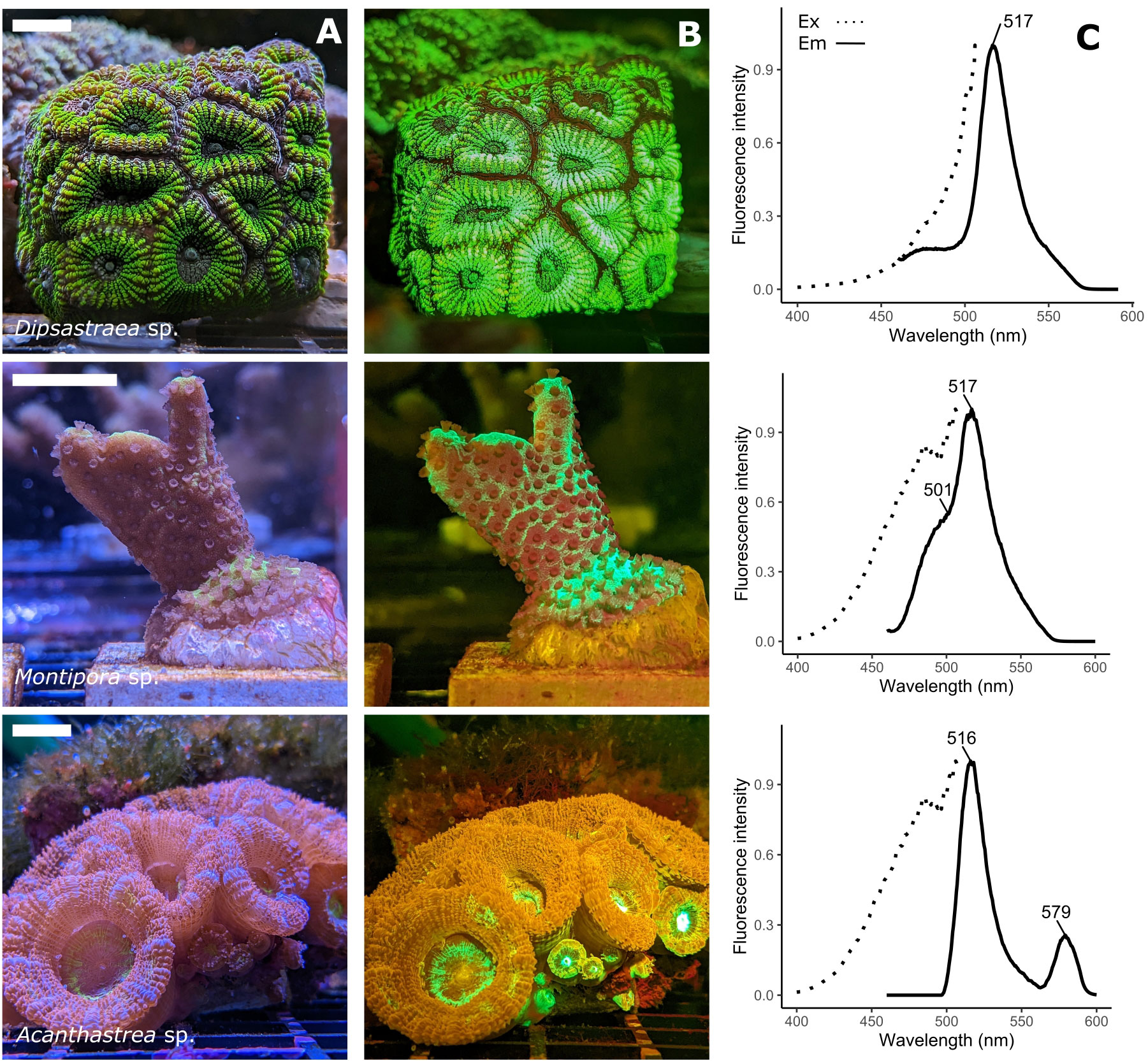This detailed scientific diagram, reminiscent of something from a science magazine or report, presents a comparative study of coral fluorescence under different lighting conditions. The diagram is organized into three vertical columns labeled A, B, and C against a white background. 

Column A features three photographs of various coral species captured in natural lighting, exhibiting their true colors with detailed textures. The corals are distinct, displaying unique natural hues from green to purple, with intricate structures.

Column B showcases the same coral species, but under UV light, which causes them to fluoresce brightly. These photographs reveal the corals glowing in vivid shades of bright green, orange, and other fluorescent colors, showing a stark contrast to their appearances in Column A.

Column C contains a series of line charts summarizing the corals' reactions to the fluorescent light. These graphs plot the wavelength against the intensity of fluorescence for each coral specimen. Each graph shows a significant peak between 500 and 550 nanometers, indicating the wavelengths at which these corals emit maximum fluorescence. Some charts include additional smaller peaks, suggesting secondary fluorescence intensities at different wavelengths.

Together, the images and graphs provide a comprehensive overview of coral fluorescence, making it a valuable visual aid for scientific analysis.